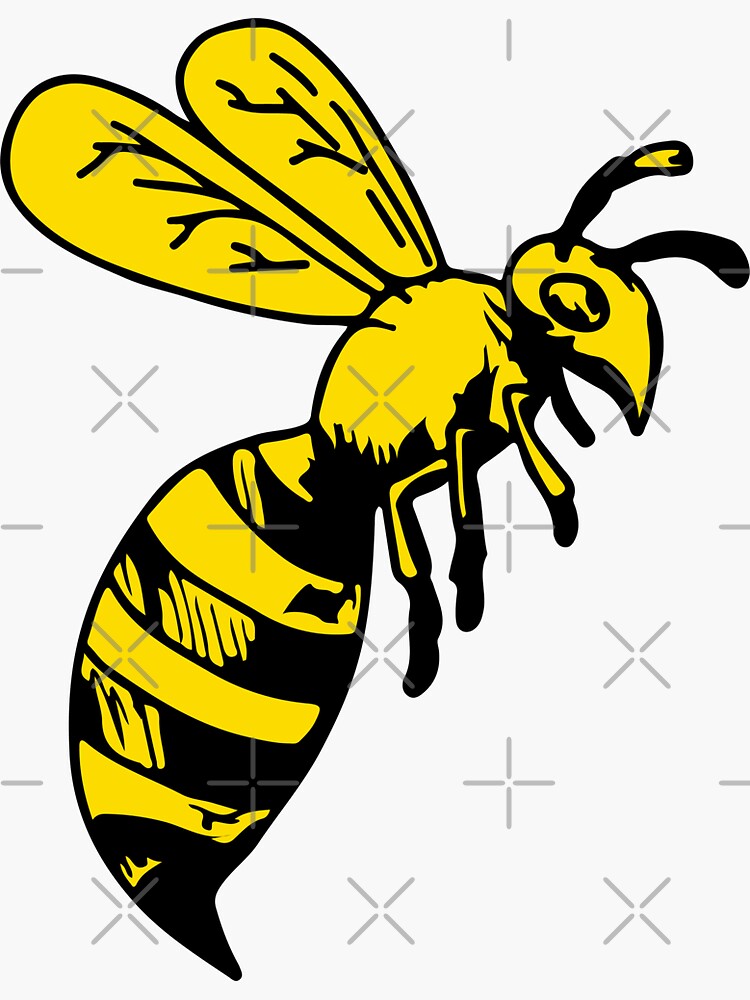The image features a highly stylized, cartoon-like drawing of a wasp highlighted by a black paintbrush texture and vivid yellow coloring. The wasp, positioned centrally, prominently displays its key anatomical features: two antennae, a pair of eyes, three visible legs, detailed wings, and a segmented body with a distinct thorax and abdomen. The abdomen is adorned with four black stripes, terminating in a noticeable black stinger. Surrounding the wasp is a white or off-white background that includes various watermarks in the form of X's, pluses, and dashes. These watermarks impose a grid-like pattern of squares across the image, indicating that the wasp graphic is still under copyright and not intended for free use. Despite the watermarks, the detailed depiction of the wasp remains clear and recognizable, with the black underbelly, yellow legs, and detailed yellow and black wings contributing to its vivid, almost primitive appearance.